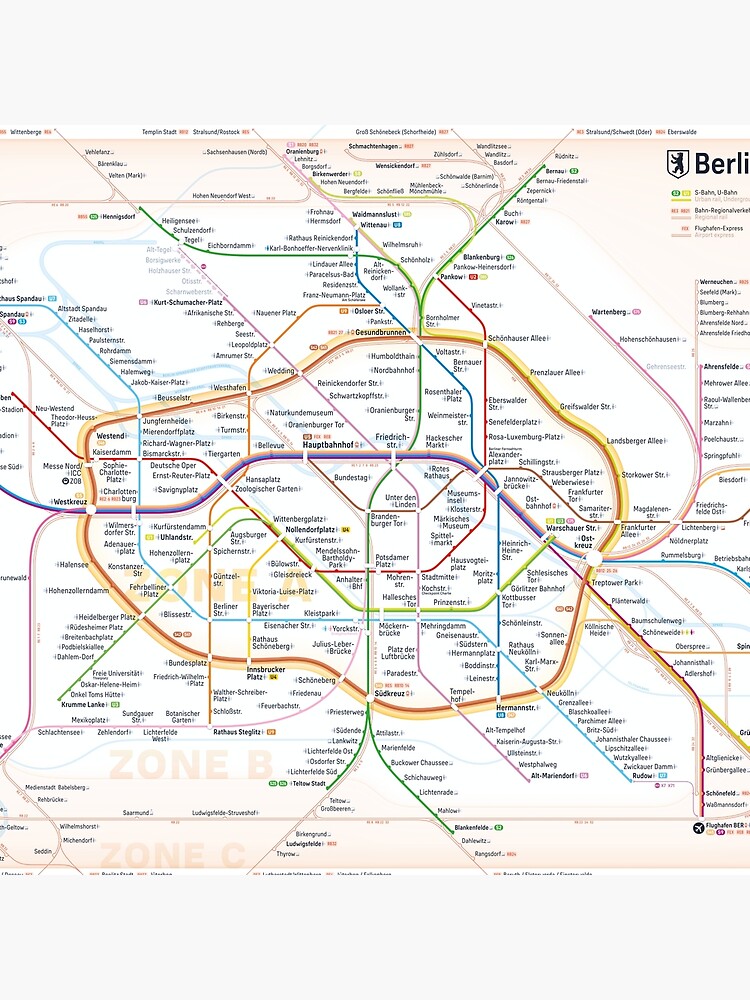The image is a detailed map of the transit system in Berlin, resembling the style of the London Underground map. It features a combination of subway and bus routes, with lines in various colors including orange, dark orange, red, green, purple, brown, and tan, all set against a light tan to white background. The multiple station stops are marked by dots and labeled with their names in German. The central area showcases a dense network of crisscrossing tracks and a circular route that encircles this hub. Lines radiate outward, extending into presumably suburban areas, with numerous stops along the way. 

A legend appears in the top right corner indicating "Berlin," although the text is partially cut off, displaying only "B-E-R-L-I." In the top left, there's a logo featuring a shield with a standing bear. The map includes faint zone markings labeled "Zone A," "Zone B," and "Zone C," likely used for fare calculation between different areas. Despite the stylized, non-geographical layout, it accurately represents the connections and routes within the Berlin transit system. The map's backdrop and multicolored lines, combined with the German text of station names, provide a comprehensive and visually engaging overview of Berlin's transit network.